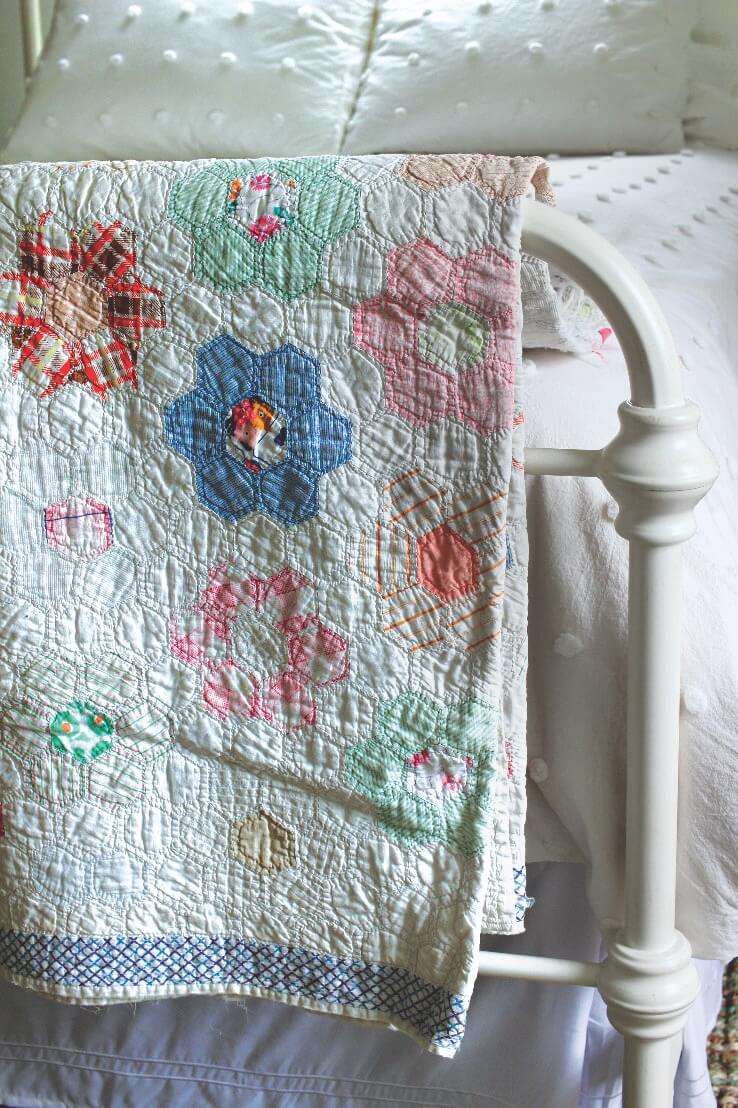The image depicts the foot of a bed with a white, possibly metal, frame painted white. The bedding consists of a white comforter adorned with rows of white dots, and two matching pillows at the head, which also feature the same dotted pattern. Tucked beneath the comforter, hints of blue bed sheets are visible. Draped over the bed frame at the foot of the bed is a quilted blanket with a colorful floral design, showcasing flowers in blue, pink, green, white, and red, including some with a plaid red and brown pattern. The overall style of the bed appears traditional and possibly intended for a child's room.